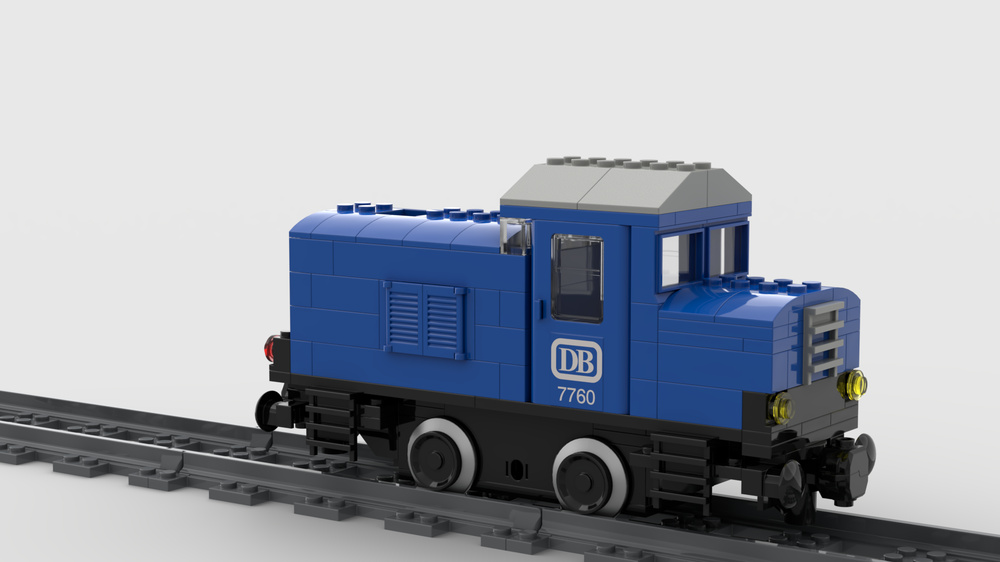This photograph, likely intended for an advertisement, features a child's toy train with a backdrop and base of plain white, reminiscent of product images one might find online. The central focus is a deep royal blue, Lego-style train segment positioned on gray plastic train tracks. This single train car, representing the locomotive, is devoid of any additional cars. The train has a gray roof, small plastic windows, and two yellow headlights at the front. The side of the car prominently displays the text "DB-7760" in white, accompanied by a white border around the "DB". The wheels of the train are a combination of black and gray plastic, and overall, the style exudes a modern, playful aesthetic.